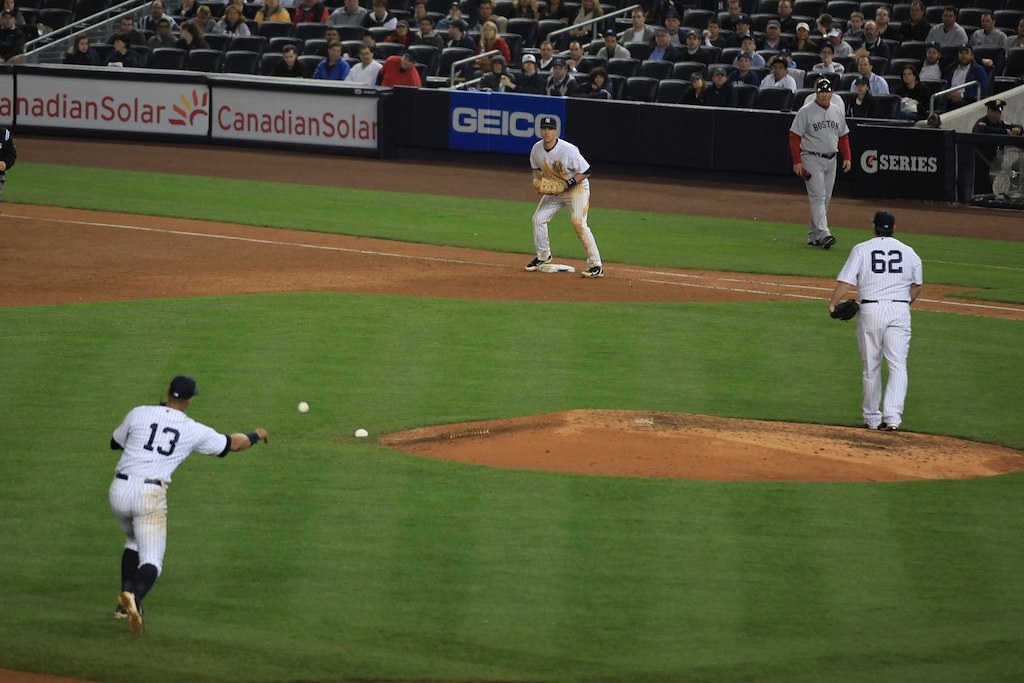This is a captivating photograph of a professional baseball game in progress, taken from a vantage point between home plate and third base, likely from the stands on the third base side. The image focuses on the infield, showcasing a pivotal moment where the third baseman, identifiable by his white uniform with knee-high black socks, a black cap, and the number 13 on his back, has just released a throw towards first base. The first baseman, dressed in the iconic New York Yankees white and black pinstripe uniform, is hunched forward, poised to catch the incoming ball with his mitt. The pitcher, standing at the edge of the brown pitcher's mound, wearing a white uniform with the number 62 on the back, and a black cap, is intently observing the play.

In the foreground, we can see the first base coach of the team in a light gray uniform with "Boston" emblazoned on the front and red sleeves, positioned off to the side near what appears to be six rows of box seats. Advertisements for Canadian Solar, GEICO, and Gatorade are visible along the outfield wall, adding to the authentic atmosphere of a high-stakes baseball game. The rectangular photograph, wider than it is tall, captures not just the intense on-field action but also the vibrant energy of the stadium environment.